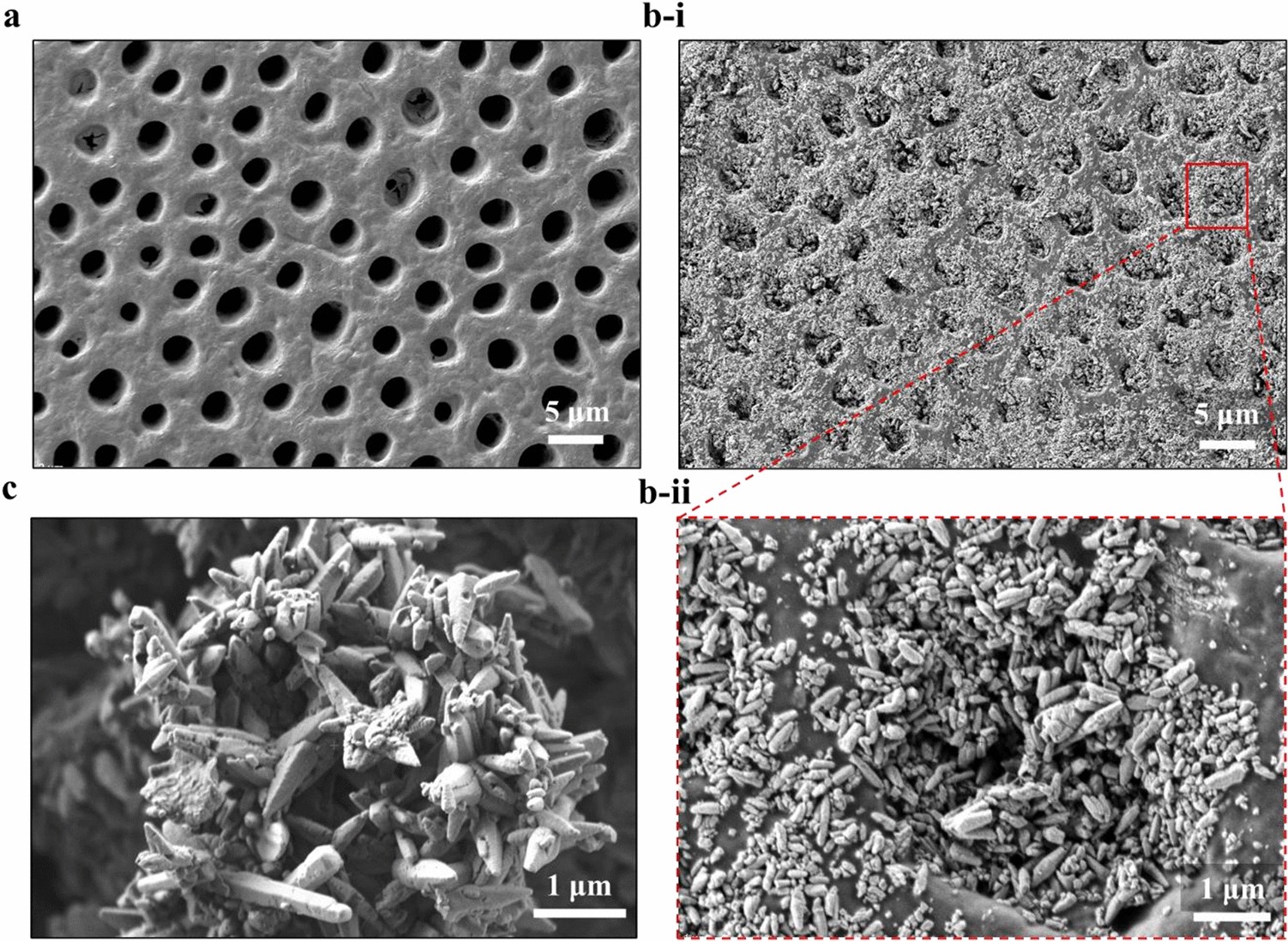The image comprises four black-and-white microscopic photographs labeled A, B1, C, and B2, arranged in a rectangular grid. The top-left image (A) reveals a textured surface with numerous holes varying in size, resembling a screen. Immediately to its right, the top-right image (B1) also depicts a similar surface but with a grainier texture and larger, dust-filled holes. These two top images are interconnected by two dotted red lines forming a triangle, directing attention towards the bottom images.

The bottom-left image (C) showcases a cluster of grayish stick-like structures, piled chaotically on top of each other, possibly resembling overgrown crystals or debris. The bottom-right image (B2) offers a close-up view of one of the holes seen in the top images, presenting a detailed look at what seems to be debris or bacterial growth, akin to tiny rice grains, clogging the pores.

Overall, the four images collectively provide an in-depth look at a porous, textured surface, first from a broader perspective and then progressively zooming in to reveal intricate details within the microscopic holes.